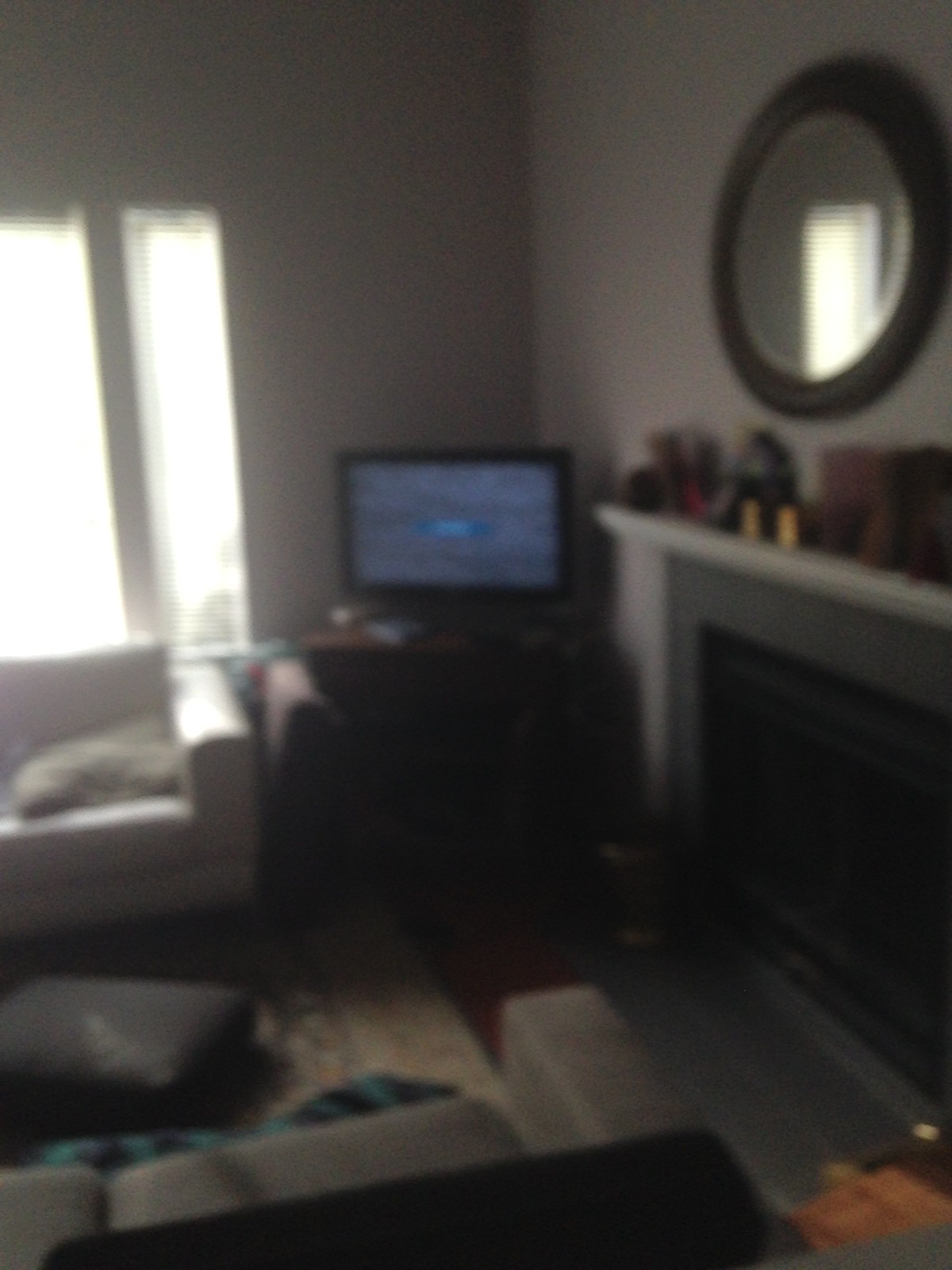The image portrays a blurry, shadowed living room scene. Central to the composition is a white-framed window emitting daylight, positioned above a white or light-reflecting couch on the left side. At the bottom left, a dark brown or gray hassock is visible, contrasting with the dark hardwood floor. Along the lower edge, you see the top of a brown two-seat sofa. The bottom right corner features a mysterious rusty brown patch. The right side of the image highlights a light gray or beige wall with a white mantle and a fireplace below it, decorated with knickknacks and perhaps visible trinkets. Above the mantle hangs a round wooden-framed mirror or possibly a clock. In the far left corner near the mantle, a small TV or computer monitor is displaying static or a default blue screen, sitting atop a brown stand. A light brown rug is placed between the two couches, adding warmth to the overall dark and blurry ambiance of the room.